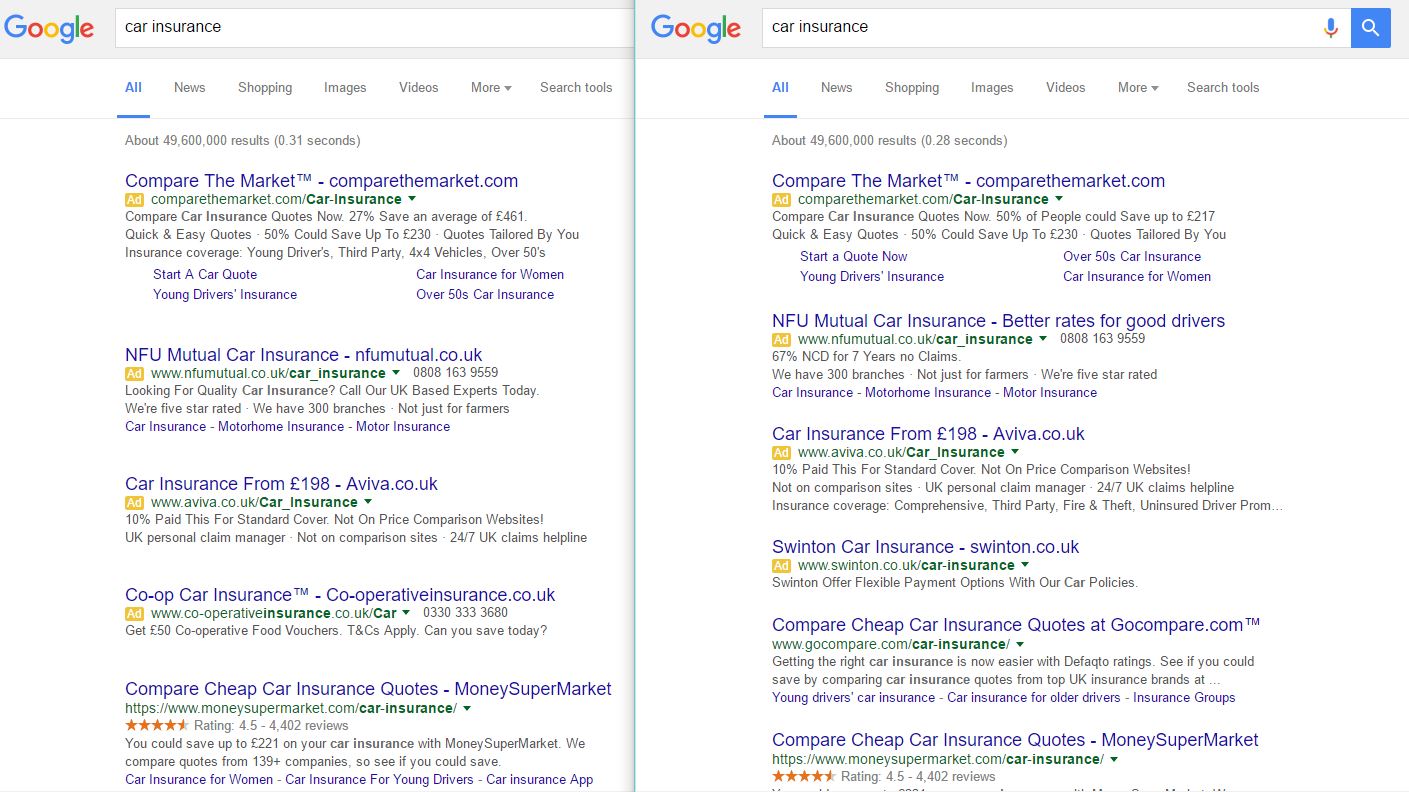The image displays two adjacent Google search results pages. On the left side, the Google search query "re-insurance" is entered into a white search box within a gray-bordered interface. The first tab, labeled "All," is highlighted in blue, while other tabs such as "News," "Shopping," "Images," "Videos," and "More search tools" are listed in black. The search yielded approximately 49,600,000 results in 0.31 seconds. 

On the right side, the search query is "Google Car Insurance," with a similar interface and a result count of approximately 49,600,000 results, but in 0.28 seconds. Both searches have several identical search results in blue with subtitles and URLs beneath each. The top result is a listing from "comparethemarket.com." The following result is from "NFUMutual.co.uk," advertising better rates for good drivers. The subsequent result, from "AVIVA.co.uk," offers car insurance starting at 198 euros. Another recurring listing is from "cooperativeinsurance.co.uk." While the left side features "Swinton.co.uk," the right side presents "GoCompare.com," both promoting the comparison of cheap car insurance quotes. The detailed search results underscore the symmetry and slight variations in search performance and results presentation.